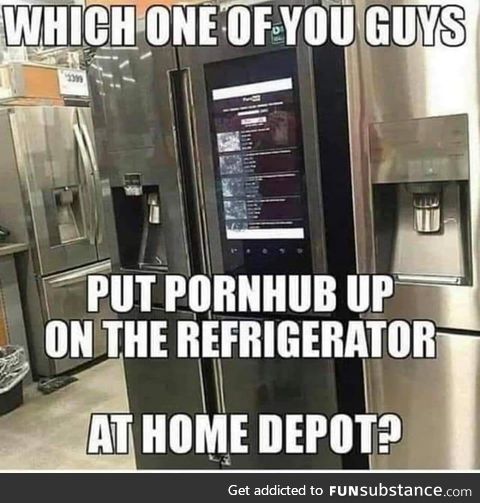The image depicts a row of stainless steel refrigerators displayed in what appears to be a Home Depot store, characterized by its indoor fluorescent lighting and tile flooring. Central to the image is a smart refrigerator with a controversial screen displaying the Pornhub website. The bright white text overlaying the image humorously reads, "Which one of you guys put Pornhub up on the refrigerator at Home Depot?" At the bottom, a black bar contains the tagline in white text, "Get addicted to funsubstance.com." The scene is further detailed by a wastebasket on the left and partial views of additional refrigerators, highlighting the store's commercial setting.